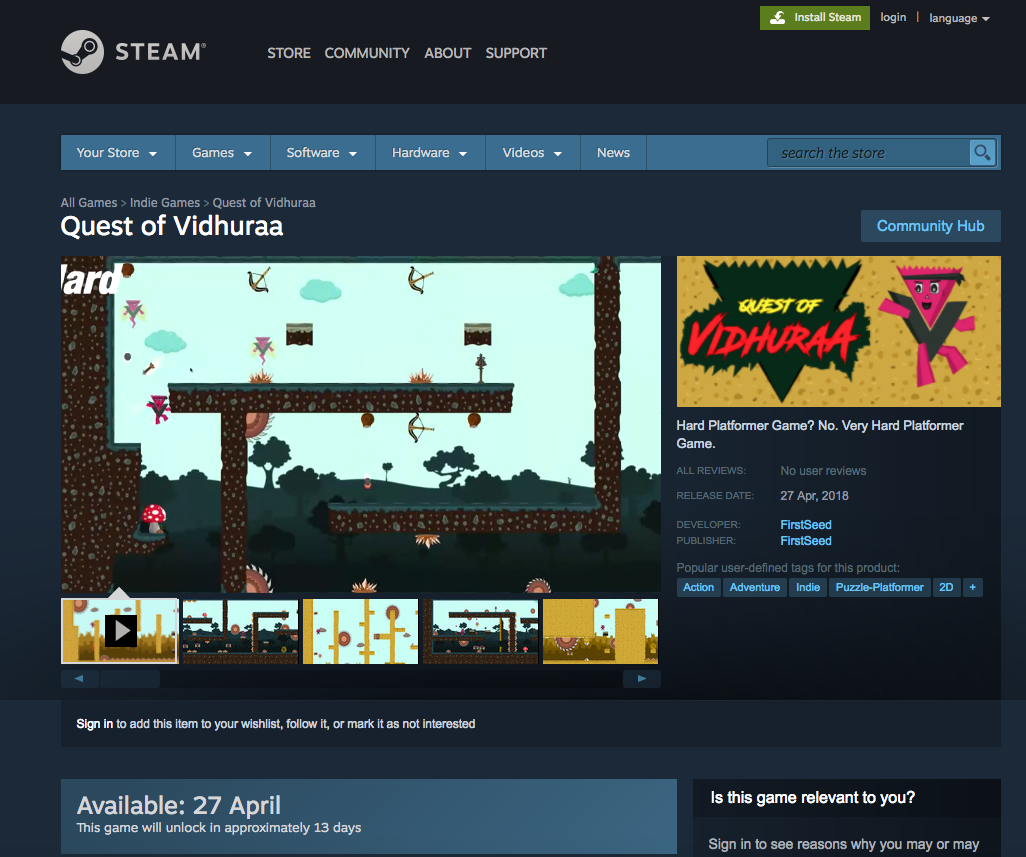The image is a screenshot taken from the Steam webpage. At the top left corner, there is a gear icon enclosed within a white circle, signifying the settings menu. Adjacent to the Steam logo, there are navigational tabs titled "Store," "Community," "About," and "Support." In the top right corner, options for "Install Steam," "Login," and a language selection drop-down menu are visible.

Below the primary navigation bar, secondary tabs are displayed, including "Your Store," "Games," "Software," "Hardware," "Videos," and "News." A search bar is located to the right, labeled "Search the store" with a magnifying glass icon at the end.

The focal point of the screen is a feature for the game "Quest of Vidura." The game's title, spelled "V-I-D-H-U-R-A-A," is prominently displayed alongside its release date, "Available April 27." The game's thumbnail showcases an environment with arrows being shot, mushrooms growing, and a landscape of brown terrain interspersed with patches of grass, suggesting a maze or adventure setting.